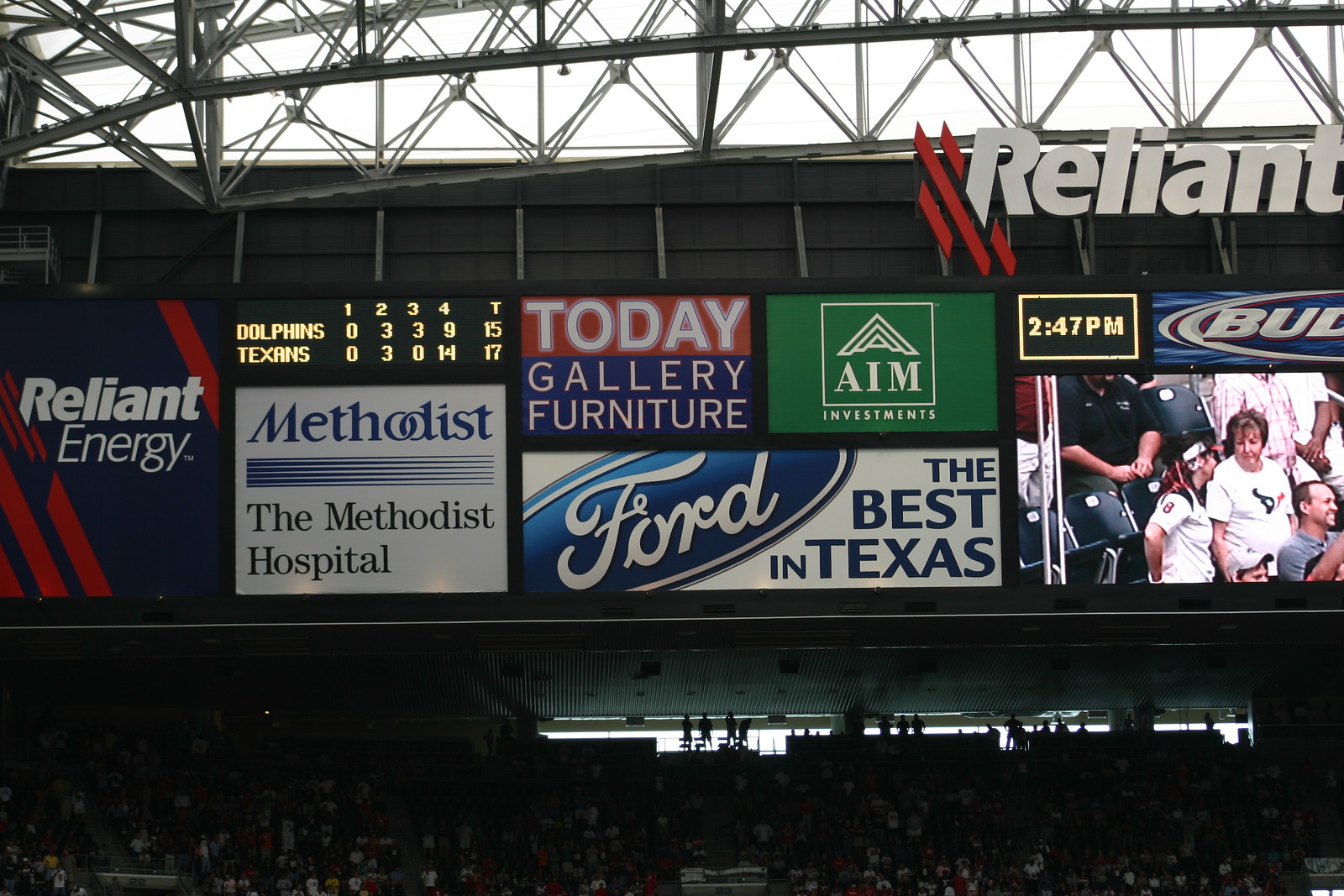The image depicts the interior of Reliant Stadium in Houston, Texas. The roof, with its lattice of white panels and dark structural lines forming a pattern of X's, spans the top of the frame. Prominently featured below is a thick gray sign reading "Reliant" with three distinct, slanted, red lines underneath.

To the left, a black sign with the same font announces "Reliant Energy," with "Energy" inscribed in thinner letters and accompanied by diagonal red lines at their corners. Adjacent to this is a digital scoreboard with the ongoing game between the Dolphins and the Texans, showing detailed scores for each quarter: 0-0 in the first, 3-3 in the second, 3-0 in the third, and 9-14 in the fourth, culminating in a current total score favoring the Texans, 17-15. 

Below the scoreboard is a white sign with the blue logo "Methodist Hospital," featuring stylized lines that thicken on the left and taper off towards the right. Next to this sign is a multi-colored ad for "Today Gallery Furniture," which displays the word "GALLERY" with spaces between each letter and "furniture" below.

Further right, a green rectangular ad for "AIM Investments" features a triangular motif above the letters "AIM." The ad below combines the Ford logo in script with the slogan "The Best in Texas." To the far right, just visible is a partial ad, presumably for Budweiser, showing "B U" in an oval blue background.

The stands below are filled with spectators, identifiable through distinct garments and positions, reflecting a lively audience intently watching the game. An additional ad in the top right corner shows "Bud Light" with the time marked at 2:47 p.m. The architectural details and vibrant advertisements together portray an engaging snapshot of a game day atmosphere at Reliant Stadium.